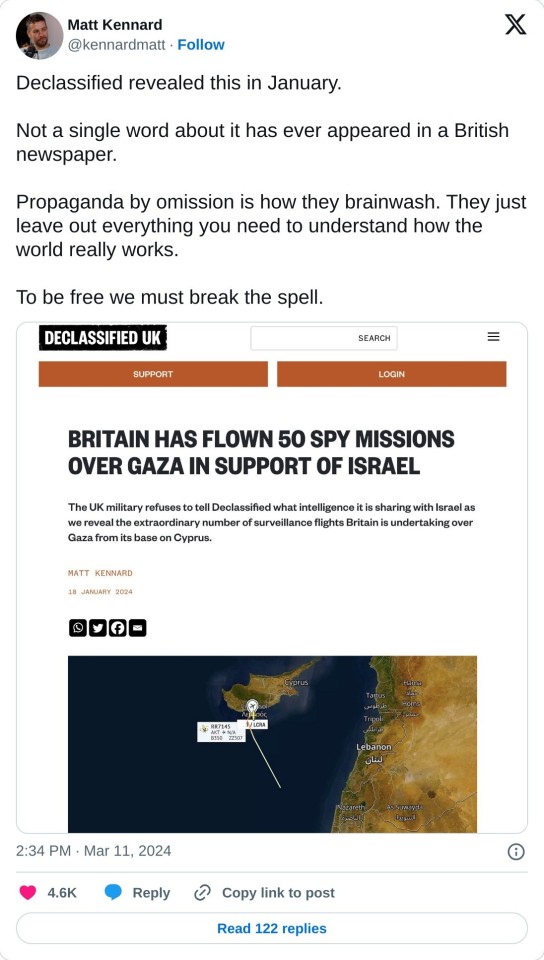A detailed screen capture from a phone displays a Twitter interface featuring a tweet by user Matt Kennard. At the top left, there is a round profile picture of a male with a beard and mustache. Beside the image, the username "Matt Kennard" is displayed in black bold font, followed by the handle "@KennardMatt" in gray, accompanied by a blue "Follow" button. In the upper right corner, an "X" icon is visible. The tweet content reads: "Declassified revealed this in January. Not a single word about it has ever appeared in a British newspaper. Propaganda by omission is how they brainwash. They just leave out everything you need to understand how the world really works. To be free, we must break the spell."

Below the tweet, there appears to be a screenshot from a website titled "Declassified UK" in black text. It features "Support" and "Log in" buttons at the top. The main article headline reads, "Britain has flown 50 spy missions over Gaza in support of Israel." At the bottom of the screen, a map is partially visible, showing a blue area representing water on the right, adjacent to a landmass.